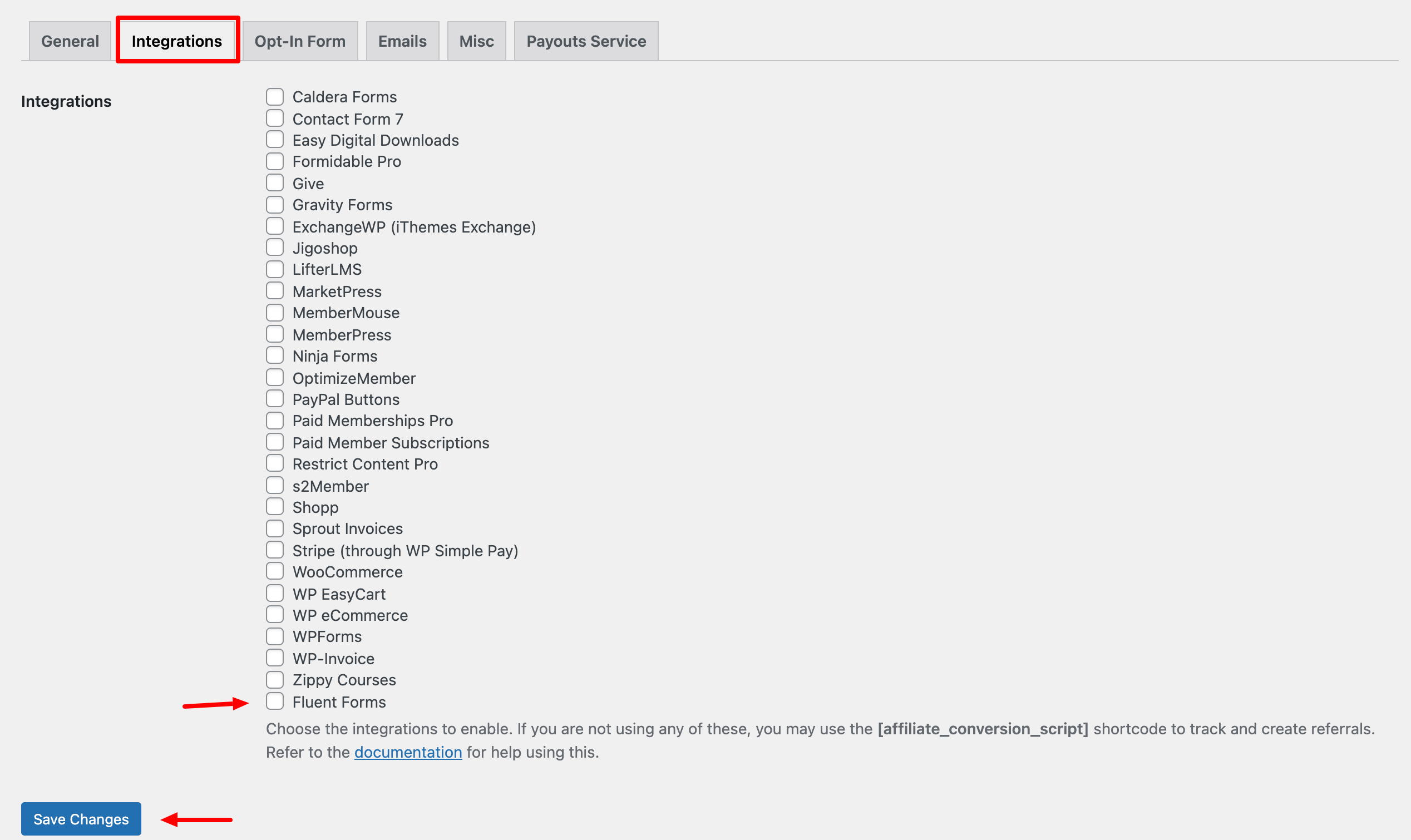A computer screen displays a gray-colored interface with various settings tabs arranged at the top, labeled as "General," "Integrations," "Opt-In Form," "Emails," "Miscellaneous," and "Payout Service." The "Integrations" tab is currently selected, revealing an extensive list of selectable integration options, including "Caldera Forms," "Contact Form 7," "Easy Digital Downloads," "Formidable Pro," "Give," "Gravity Forms," "iThemes Exchange," "LifterLMS," "MarketPress," "MemberMouse," "MemberPress," "Ninja Forms," "OptimizeMember," "PayPal Buttons," "Paid Memberships Pro," "Paid Member Subscriptions," "Restrict Content Pro," "s2Member," "Sprout Invoices," "Stripe," "WooCommerce," "WP EasyCart," "WP eCommerce," "WP Forms," "WP Invoice," "Zippy Courses," and "Fluid Forms." A user instruction at the bottom advises to "choose the integrations to enable." It also mentions that if none of these are in use, one may utilize an affiliate conversion script shortcode to track and create referrals, with a reference to the documentation or help section for further assistance. At the bottom of the screen, there is a visible "Save Changes" button.